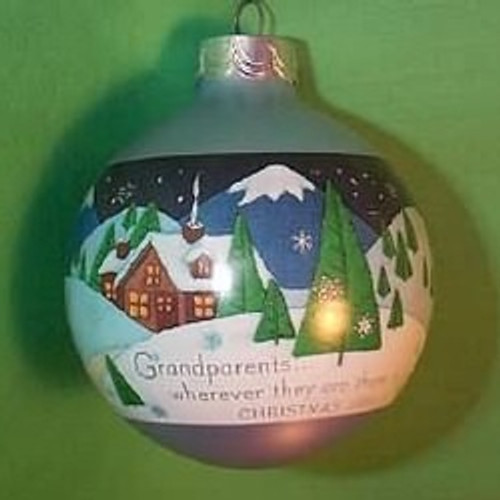The image depicts a slightly blurry, round Christmas ornament set against a medium-toned green square background. The ornament, silver in color, features a bright gold cap with a hook for hanging. Prominently painted on the front is a festive holiday scene: a small brown house with golden-lit windows and smoke curling from its chimney, nestled amidst snowy hills. Green, triangle-shaped pine trees dot the landscape, and a mountain rises in the background under a winter sky dotted with snowflakes. At the bottom of the scene, partially legible text reads, "grandparents wherever they are Christmas." The ornament's reflective surface casts subtle shadows onto the green surface beneath it, emphasizing its spherical shape.